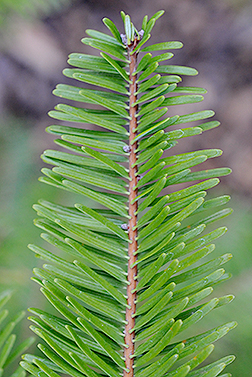This close-up image captures the end of a branch from an evergreen tree, specifically identified as an Abies homolepis, or Nikko Fir. The central feature is a slender, brown, woody branch that runs vertically through the frame. Radiating from this central branch are numerous tiny, slender, long evergreen leaves that are uniform in shape, resembling elongated rectangles. These leaves extend outwards in all directions, giving the impression that the small limb is impressively supporting a dense cluster of foliage. The branch culminates in several small buds, hinting at the future growth of pine cones. The background is a blur of indistinct brown hues, possibly soil or a rock formation, emphasizing the photographer's intent to maintain sharp focus on the intricate details of the limb. The overall setting appears forest-like, with a subdued lighting that suggests an overcast day.